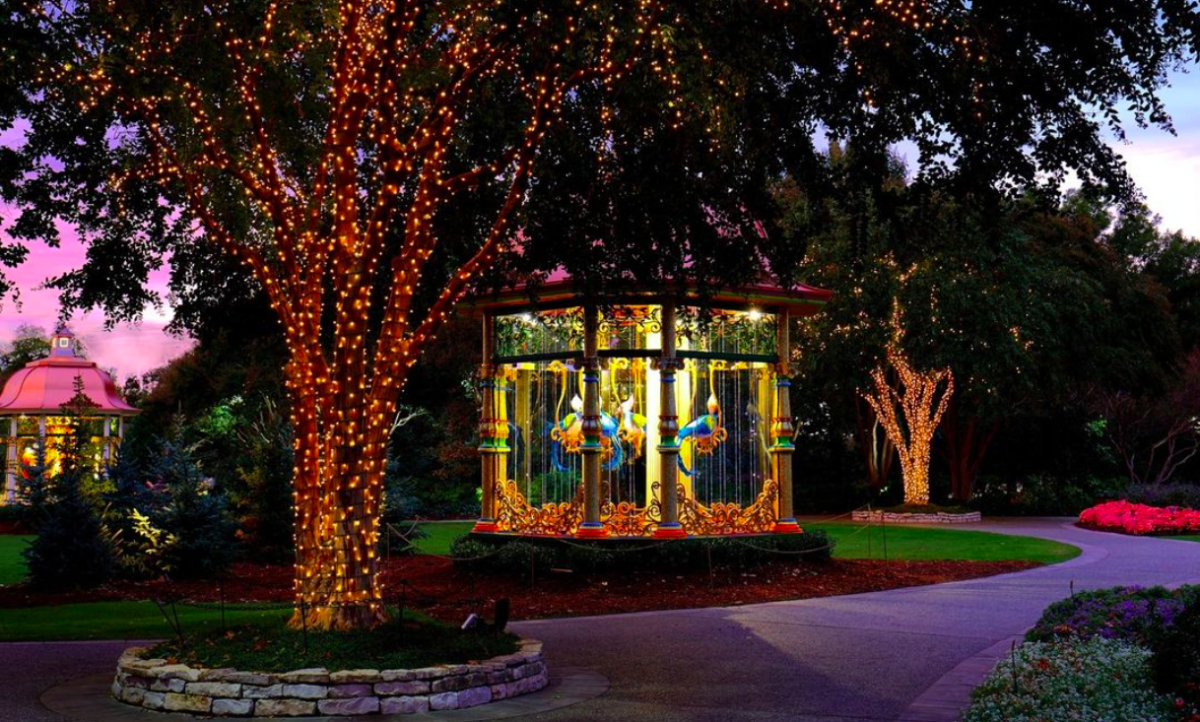The photograph captures a picturesque scene of a well-manicured park or public garden at sunset, with a beautifully decorated, festive atmosphere. One side of the sky shows a deep purple transitioning to a deep pink hue, while the other side remains a soft blue with scattered clouds, creating a serene backdrop. The park is adorned with trees whose trunks and lower branches are wrapped meticulously in thick layers of Christmas lights. Some lights even extend to the leaves, casting a magical glow on the surroundings. 

In the foreground, a large tree stands prominently, its branches sprawling and decorated with fairy lights that enhance the enchanting ambiance. The scene is dotted with bright pink, white, and purple flowers, adding bursts of color to the lush, well-maintained lawn. Stone-paved pathways wind through the park, curving gently and leading to various features.

Notably, there are two gazebo-like structures, or pergolas, illuminated from within. The main gazebo, closest to the center, is open on all sides with a small, possibly pink roof. It appears to house suspended, ornate sculptures, perhaps resembling peacocks or fish in blue and gold hues, giving it an enigmatic charm. The second pergola is toward the back, partly obscured by small trees, but it also seems to contain similar decorative elements.

Additionally, a carousel featuring rideable peacocks adds a whimsical touch to this delightful space. The scene suggests an evening event at this public garden, creating a captivating and festive environment enhanced by the interplay of natural and artificial lights.